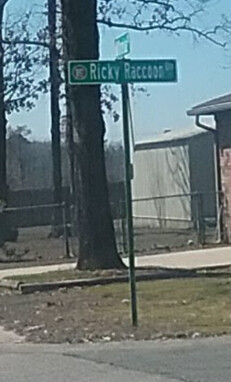The photograph captures a pair of green, rectangular street signs mounted on a metal pole. The top sign is angled away, making its text unreadable, while the bottom sign clearly reads "Recky Raccoon" in white font. The scene is set in a well-groomed yard, with short grass interspersed with dirt and rocks. In the background, tree trunks are visible, adding a touch of nature to the image. On the right side, the back end of a brown brick house and a light gray or white shed are discernible. In the foreground, a gray road cuts across the scene, completing the suburban setting.